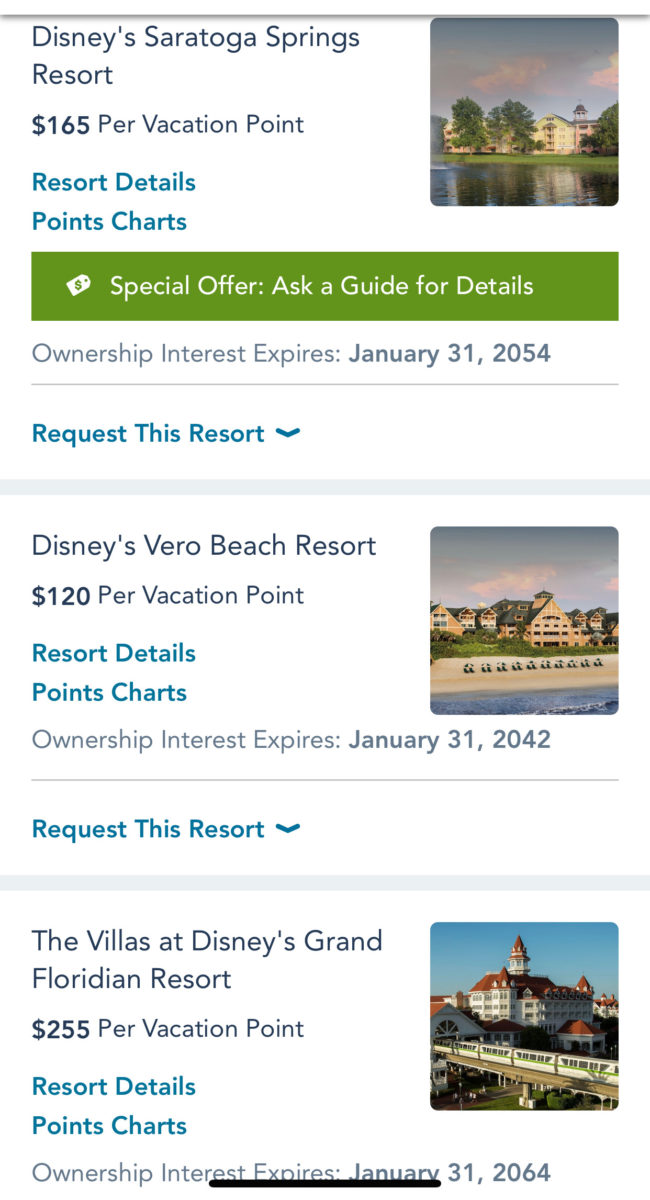The image depicts a mobile-friendly travel webpage, focusing on Disney vacation resorts. It features a comprehensive list of resort options, each accompanied by pertinent details and prices. The screen is formatted vertically, resembling a typical phone display, though no phone icons are visible.

At the top of the page, there is a segment detailing “Disney Saratoga Springs” resort, priced at $165 per vacation point. This section includes resort details, point charts, special offers, and an option to request more information by contacting a guide. Users can select this resort via a dropdown menu. Additionally, there’s a mention that ownership interest expires on January 31st, 2054, indicating that this might be a timeshare option.

Next, the webpage highlights the “Disney Vero Beach Resort,” available for $120 per vacation point. This entry mirrors the first one, providing resort details, point charts, and the ownership interest expiration date of January 31st, 2042. Users also have the option to request this resort.

Lastly, the site features “The Villas at Disney Grand Floridian Resort,” at $255 per vacation point. Similar to the others, it offers links to resort details and point charts.

Each resort listing is accompanied by a thumbnail image of the respective property, providing a visual reference for users. This suggests the webpage not only facilitates vacation bookings but also allows users to accumulate and use vacation points for additional benefits.